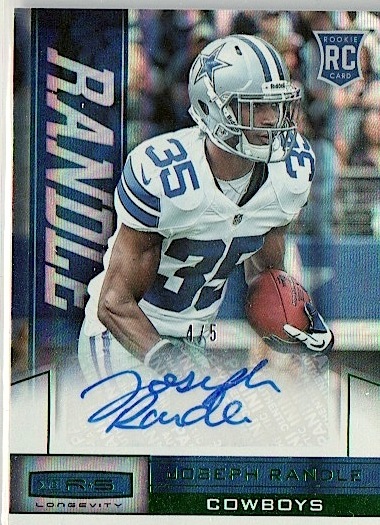This is a color photograph of a football trading card featuring Joseph Randall, a player for the Dallas Cowboys. At the center of the card, Randall is depicted in action, holding a football while wearing a blue and white uniform with the number 35 and a silver helmet displaying the Cowboys logo. The background shows an out-of-focus crowd, suggesting a lively game atmosphere. The upper right-hand corner of the card features a blue "RC Rookie Card" logo. Along the left-hand side, the name "Randall" is printed vertically. Below the main image, there is a blue signature on a white background that reads "Joseph Randall." Additionally, at the bottom of the card, "Joseph Randall" is printed again, along with the word "Cowboys" in white text on a black band. On the bottom left, there's an "RS Longevity" logo. This detailed card showcases Joseph Randall as a promising rookie for the Cowboys.